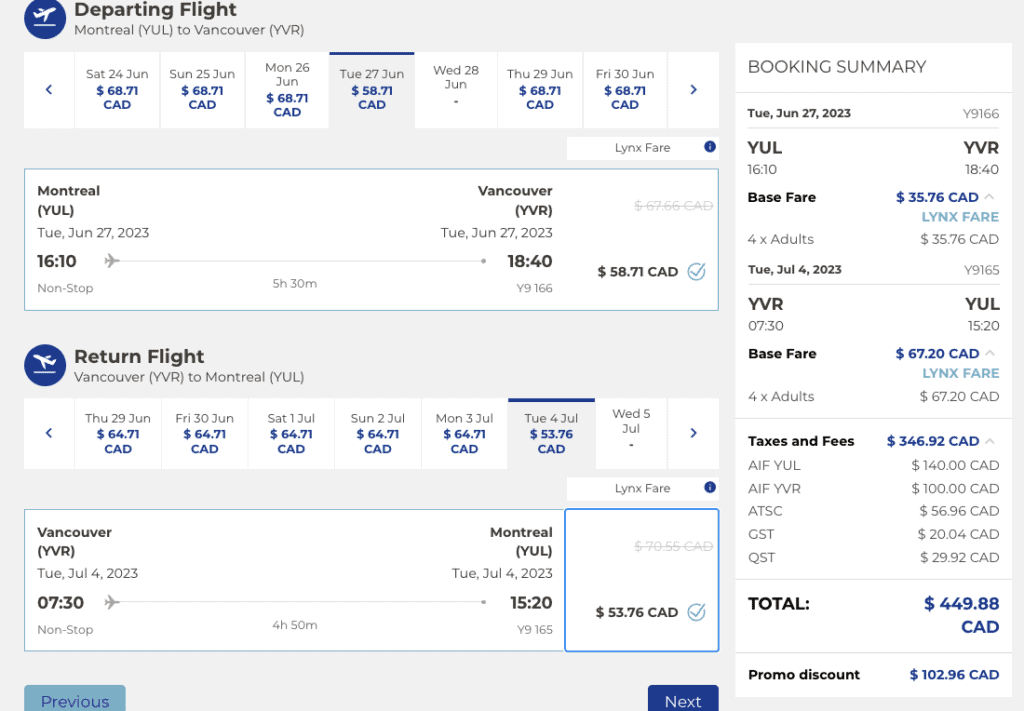The image features a website interface displaying a series of departing flights from Montreal to Vancouver. At the very top, there's a line of text that reads "Departing Flights: Montreal to Vancouver," accompanied by a small airplane icon to the left. Moving horizontally, the dates are listed as Saturday, June 24th, Sunday, June 25th, Monday, June 26th, and so on, until Friday, June 30th. The flight price for each of these dates is consistently $68.71.

On the left side of the interface, a white rectangle highlights a specific flight on Tuesday, June 27th, 2023. A gray line, adorned with an airplane icon, extends across the screen, detailing two flight times: 16:10 (4:10 PM) and 18:40 (6:40 PM), priced at $58.71.

Below this section, another small airplane icon introduces the return flights. These flights span Thursday, June 29th, to Friday, July 5th. A notable fare on Tuesday is $53.76, while the price for all other days is $64.71.

Further details include specific flights from Vancouver on July 4th at 07:30 AM and 15:20 (3:20 PM), both priced at $53.76.

To the right of the screen, there's a booking summary. This summary recaps all selected flights, breaking down the costs into base fare, taxes, and fees, culminating in a total of $449.88. Additionally, a promotional discount of $102.96 is applied.